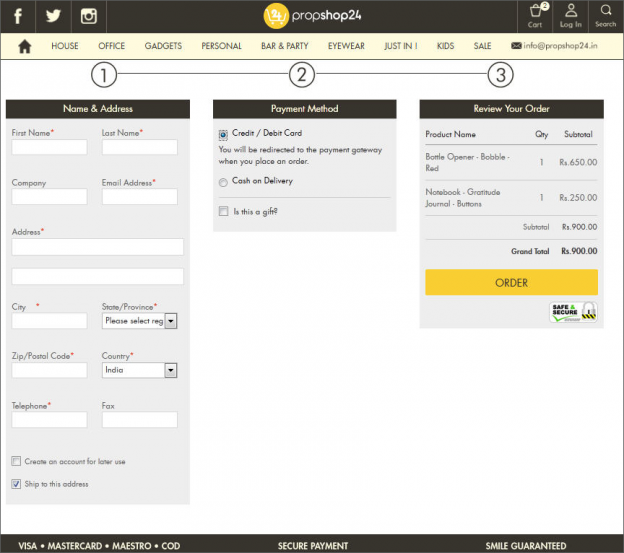The image features a multi-section interface that appears to be a webpage, divided into various functional areas with distinct colors and shapes. The top section features a dark gray background on the left with a beige color on the right. Within this area, there are recognizable social media logos: the Facebook "F" logo, the Twitter bird, and the Instagram camera icon. 

As you move across this top section, there is a prominent yellow circle containing a white heart icon and the number "24" inside. This is followed by the text "Prop Shop 24." Continuing right, there is an icon of a card with a circle, displaying the number "2" inside it. Nearby, there is a "Log in" link and a search bar iconified with a magnifying lens above it.

The background of the interface transitions into a very light yellow hue. Below, matching the top section's dark gray color, there is a navigation menu with labeled icons: "House," "Office," "Gadgets," "Personal," "Bar and Party." 

In a subsection titled "Justin," there's a prompt inviting sellers to contact via "info@propshop.in". 

Further down, there are three consecutively numbered circles in white and dark gray colors, titled "1, 2, 3." 

1. The first section, titled "Name and Address," contains fields for inputting personal information including first name, last name, company, email address, physical address, city, zip code, telephone, and dropdown menus to select state and country.

2. The second section, titled "Payment Method," offers options for transactions: "Credit Card/Debit Card," which notes that you will be directed to a payment gateway upon placing an order, and "Cash on Delivery." It also inquires, "Is this a gift?"

3. The third section lists order details with product names: "Bottle Opener," "Bubble Red," "Notebook," "Gratitude Journal," "Buttons." The total price is specified as "RS 900.00," although the exact currency is unclear.

This organized layout provides a comprehensive snapshot of the page, offering easy navigation and clear instructions for the user.